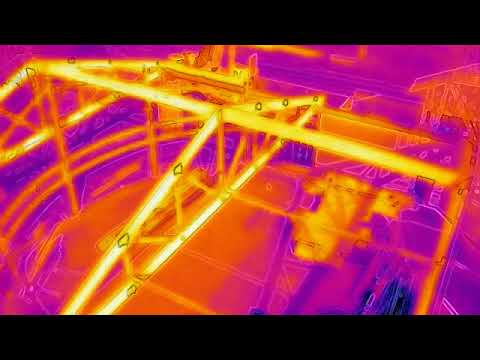The image appears to be an infrared or thermal photograph, dominated by vibrant hues of purple, orange, yellow, and pink. It seems to depict an open structure, possibly the skeletal beams of a house or perhaps a bridge under construction, bathed in differing temperatures. The triangular roof trusses or beams are prominently glowing yellow, indicating higher temperatures, while cooler areas are cast in purples and darker oranges. The photograph is letterboxed with black bars at the top and bottom. In the upper right, there seems to be an outline of what could be a barn or storage shed, adding a sense of depth and context to the structure. On the left of the image, below the triangular beams, an orange circular area is visible, further highlighting the temperature variance throughout the structure.